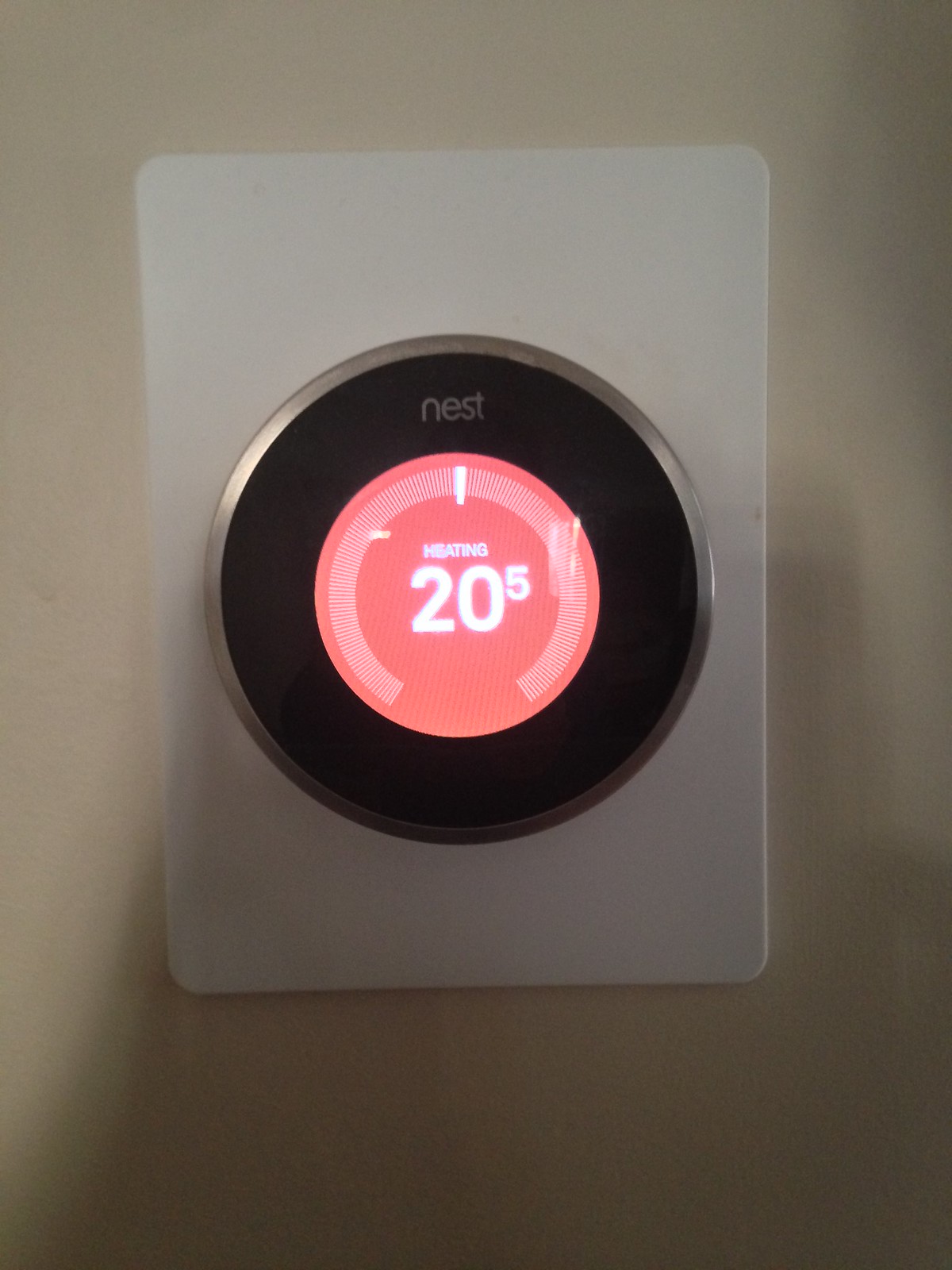The image depicts a high-quality photograph of a Nest thermostat mounted on an off-white wall. The thermostat itself is a sleek, white rectangular device with rounded edges and features a distinctive silver frame. At the center, there is a black circular display with the word "Nest" at the top. Prominently displayed in the middle of this circle is a red indicator, showing the current heating status with the temperature set to 20 degrees. Adjacent to the 20, there's a smaller number 5, which likely indicates some additional parameter. Surrounding the red circle are various lines resembling a gauge, suggesting that the device can be manually adjusted by turning it. In the background, a shadow reveals that someone is holding up their phone to take the photo, capturing both the thermostat and its sleek, modern design against the wall.